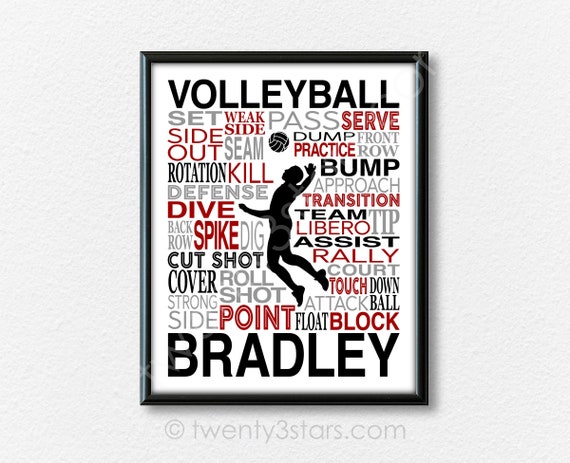This photograph features a decorative wall hanging presented within a sleek black frame, mounted against a white speckled wall. Below the hanging, a discreet gray watermark reading "20numberthreeStars.com" is visible. The central element of this artwork is a stylized black cartoon figure in mid-air, poised to spike a volleyball with dynamic energy. The design itself employs a bold color palette and text styles in shades of black, gray, and red, creating a visually striking composition.

The upper portion prominently displays the word "Volleyball" in a bold black font, while the bottom showcases the name "Bradley" also in black. Surrounding the central figure are numerous terms related to volleyball, interspersed throughout the artwork in varying fonts and colors, adding texture and emphasis. Words like "pass, serve, bump, spike, cut shot, cover, point, float, block, attack, and ball" highlight key aspects of the sport, with many other volleyball terms layered throughout the piece, contributing to its richness and detail.

The interplay of font variations and colors not only enhances the aesthetic appeal but also emphasizes the passion and dynamism associated with volleyball, making this wall hanging both a visually appealing and meaningful tribute to the sport.